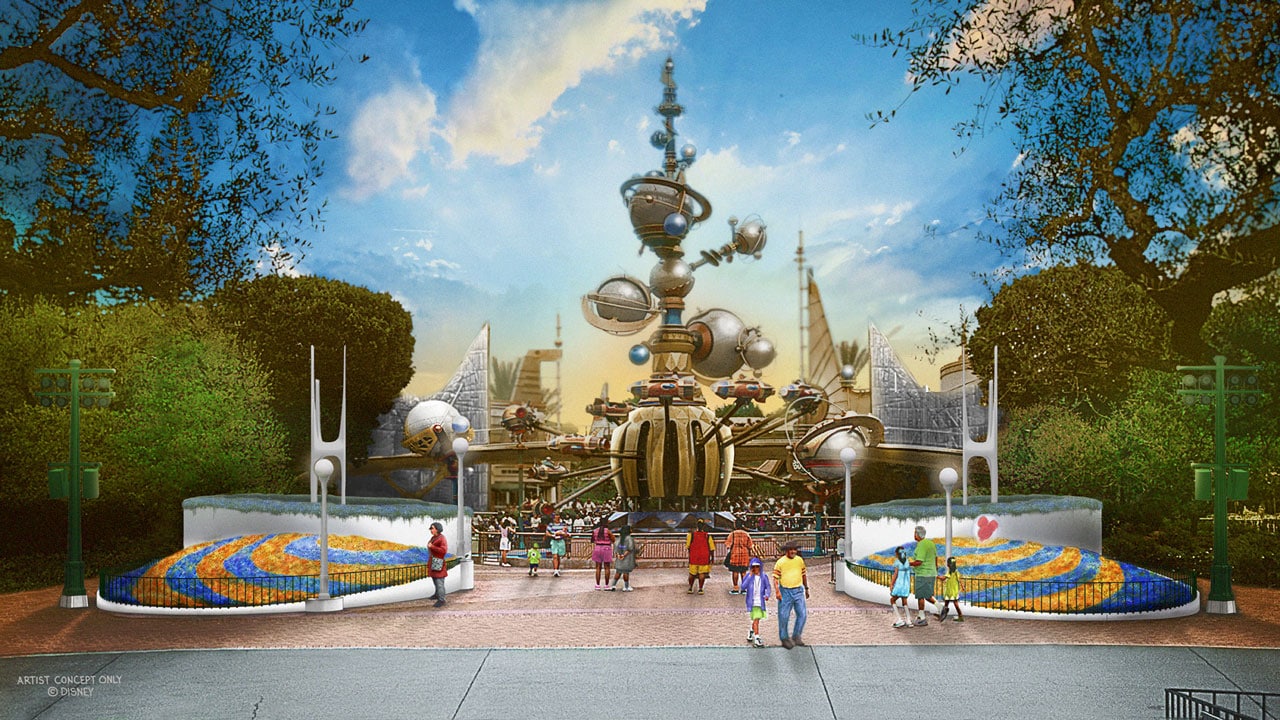The image is an artist's rendition of a futuristic theme park attraction, presented in a horizontally aligned rectangular depiction. At the bottom left corner, white text reads, "Artist Concept Only. Copyright Disney." The bottom area features large square sections of dark gray concrete resembling a road or walkway. Above this, a paved brown pedestrian walkway leads into the park. Central to the image is a black gate flanked by circular landscapes with low white walls, adorned with yellow, blue, and orange striped flowers.

Multiple visitors are strolling towards the park’s entrance, enhancing the lively atmosphere. Dominating the center of the illustration is a towering structure, characterized by a series of circular objects and smaller hanging circles that resemble planets orbiting a futuristic metal tower. This structure, with its metallic finish and gold hues, culminates in a steeple-like tip. The background features a blue sky with light, feathery clouds and trees on both the left and right sides. The detailed and vibrant design captures a dynamic, otherworldly attraction within a Disney theme park.